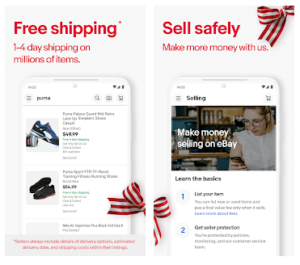In the image, there is detailed promotional content against a gray background. On the left side of the image, red text reads, "Free Shipping: 1 to 4 day shipping on millions of items." Beneath this text are two product listings; the top listing features shoes, while the bottom listing also displays shoes, specifically black ones. However, the information accompanying these listings is too small to be discerned.

On the right side, there is a marketing message in red text that states, "Sell safely, make more money with us," accentuated by a ribbon in the top right corner. Below this text, a smartphone screen displays a webpage with the headline, "Make money selling on eBay," and features an image of a woman inside her home. Further below, there's a very small two-step process explanation with a ribbon on its left side. The image concludes succinctly, thanking the viewers.